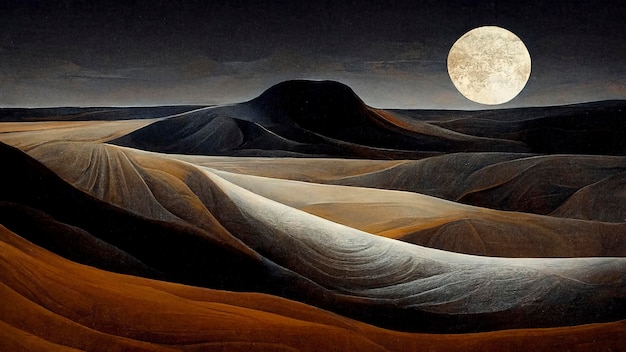The image portrays a digital screenshot of a captivating piece of artwork that illustrates an evening scene in a desert, dominated by a blood moon rising over a rolling mountain range. The large moon, positioned in the top right corner, casts an ethereal white glow that contrasts starkly with the darkening sky, which transitions from a dark gray near the horizon to almost black at the top. The desert landscape is an intricate tapestry of sand dunes and mountains, resembling the intricate patterns of woodgrain with shades ranging from copper red to deep black, tan, beige, and stone-like colors. The dunes and mountains cascade downwards and extend well into the distance, creating a sense of depth and vastness. Notably, there is a tall mountain situated about three-quarters into the distance, standing as the highest peak in the scene. This artwork effectively captures the quiet majesty and solitude of a desert night under a hauntingly beautiful moon.